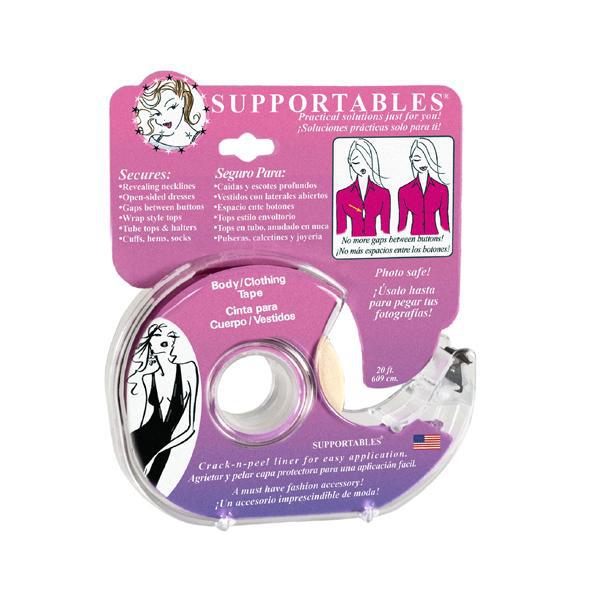The image depicts an advertisement for "Supportables" body clothing tape designed for securing women's clothing and preventing wardrobe malfunctions. The packaging is primarily pink and purple with white text and includes both English and Spanish descriptions. At the top, it prominently features the brand name "Supportables" along with the tagline "Practical Solutions Just For You!" and its Spanish equivalent "Soluciones Prácticas Sólo Para Ti!"

To the upper left of the package, there is an illustration of a blonde woman with makeup and red lipstick, making a flirty face, surrounded by stars within a circle. Below this image, the packaging lists the various uses for the tape including, but not limited to, securing revealing necklines, open-sided dresses, gaps between buttons, wrap-style tops, tube tops, halters, cuffs, hems, and socks, with the same information provided in Spanish on the right side.

The center of the graphic includes side-by-side illustrations demonstrating the tape's effectiveness. The left image shows the woman wearing a red blouse with a gap between the buttons, while the right image showcases the same blouse perfectly secured with no gaps using the tape. Another image displays the woman in a tight black dress with revealing cleavage, further emphasizing how the tape can maintain modesty and secure clothing.

The actual roll of body tape is portrayed within the package, resembling a scotch tape roll with a plastic spool and cutter. The roll also features the same blonde woman in a black dress, illustrating the product in use. Additional text indicates that the tape is Photosafe, ensuring it remains discreet and effective in any situation. A small USA flag is also visible, hinting at the product's origin.